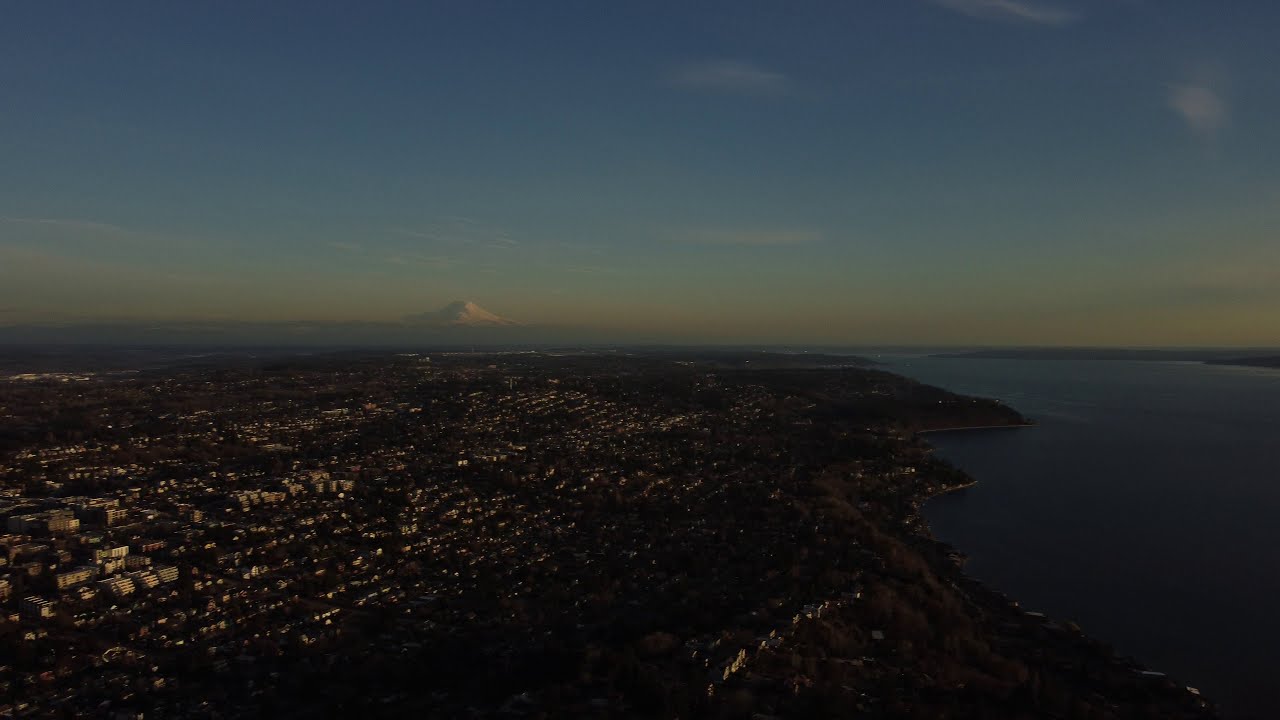The image is a color photograph taken at dusk or night, captured from a high vantage point, potentially by a drone. It is presented in landscape orientation, reminiscent of a high-definition television with its wider-than-tall aspect ratio. The scene overlooks a town or small city situated by the sea, viewed from above, casting the town in deep shadow with the setting sun barely illuminating the landscape. 

The land extends about two-thirds of the way across the image from left to right and occupies about half of the photograph's height. Scattered low-level buildings and clusters of houses are faintly visible in the foreground, their details muted by the encroaching darkness. The sea is prominently featured on the right side of the image, wrapping around the land's edge, creating a natural curve that leads the eye to the distant horizon. 

In the distance, a snowy mountain peak stands tall, positioned slightly left of center, against a backdrop of a twilight sky. This sky transitions from dark blue at the top to lighter blue with a hint of pale orange near the horizon. The photograph embodies a sense of realism and quiet beauty, capturing the serene and slightly eerie transition from day to night over this coastal town.